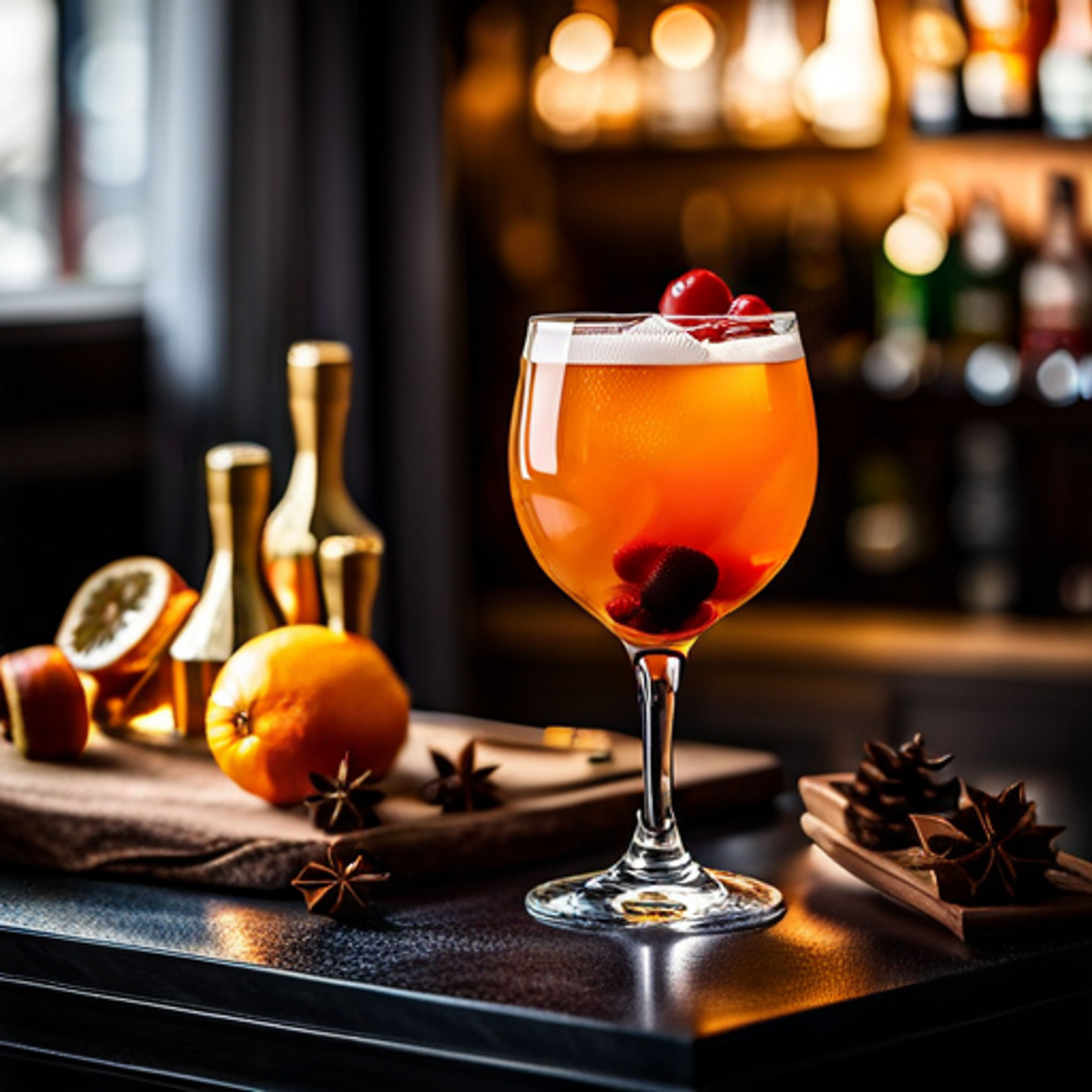In this indoor image, likely taken near a bar, a vibrant scene unfolds. The background is slightly blurred but discernible, revealing a bar-like setting with shiny glass objects, including several bottles and a green ball. One bottle has a distinctive white and red label. There's also a long gray curtain and a window on the left side, with light streaming in. This mix of greens and burgundy contributes to the overall atmosphere.

In the foreground, a black surface hosts a wooden table adorned with various items, most prominently a brown cutting board. On the cutting board rests an uncut orange, a pair of small golden brass containers, some star anise, and what appears to be a clock. To the right, a small brown object is situated.

The central focus of the image is a clear wine glass containing a vibrant orange liquid with foam on top. Suspended within the glass is a cherry, while two or three more cherries float above the foam. Bubbles emerge from the dissolving elements within the drink. The well-lit scene makes the reflection of the window visible on the glass, enhancing the rich details. The overall color theme leans towards darker browns, adding warmth and depth to the image.